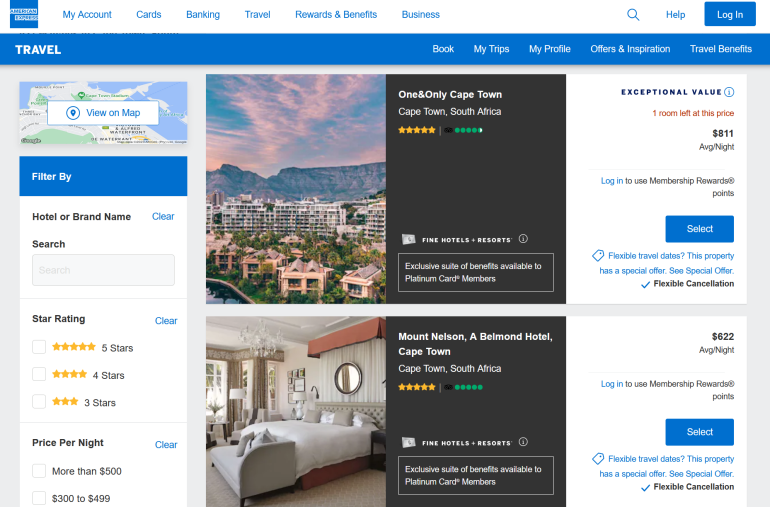The image depicts a detailed page from the American Express website. At the top, the familiar American Express logo in blue is prominently displayed, accompanied by an array of navigational filters including My Account, Cards, Banking, Travel, Rewards and Benefits, and Business. A search button, a help option, and a blue login button are also visible.

The main focus of the page is the Travel section, showcasing various subsections such as Book, My Trips, My Profile, Offers and Inspiration, and Travel Benefits. There is also a map section labeled "View on Map" that features a sophisticated filter system. Users can filter their search results by hotel or brand name, star rating, or price per night through a clearly marked search box and options.

The search results display several images. One notable entry is 'The One and Only Cape Town' in Cape Town, South Africa. The image captures the stunning view of a mountain backdrop alongside a cluster of resort buildings. Another entry features 'Mount Nelson, a Belmond Hotel,' also located in Cape Town, which is showcased with a star rating and a TripAdvisor rating. The image of Mount Nelson offers a glimpse into a spacious hotel room with additional seating arrangements.

Pricing details are provided, with 'The One and Only Cape Town' listed at $811 per night, noted as exceptional value and highlighting that only one room is left at this price. Meanwhile, 'Mount Nelson, a Belmond Hotel' is priced at an average of $622 per night. A login option and information on flexible travel dates and special offers are also mentioned, enhancing the utility and attractiveness of the travel booking experience.